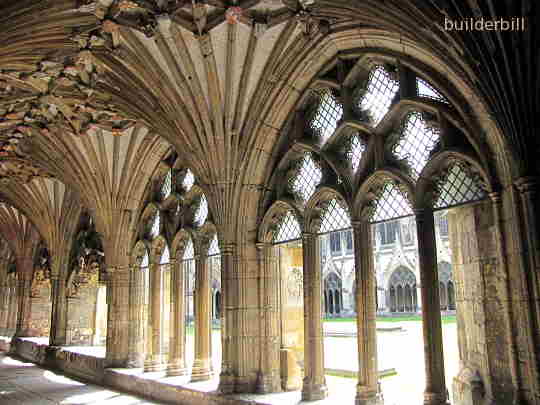The photograph captures an elaborately designed open hallway or cloister within an old stone building, potentially of a historical church or university. The architecture, reminiscent of Greek or Roman design with a hint of gothic elements, features large, decorative stone columns supporting towering, pointed arches. These arches rise into a fan-shaped, intricately carved ceiling. On the right side, the columns frame an open view leading to a sunlit courtyard, visible through tall, narrow windows adorned with triangular panes of glass set in fleur-de-lis stone carvings. The ground is paved with cement, adding to the structure’s ancient ambiance. Across the courtyard, there is a facing building of similar architectural style, enhancing the scene’s symmetrical beauty and historic charm. Grass within the courtyard adds a touch of nature to this majestic and timeless stone corridor.